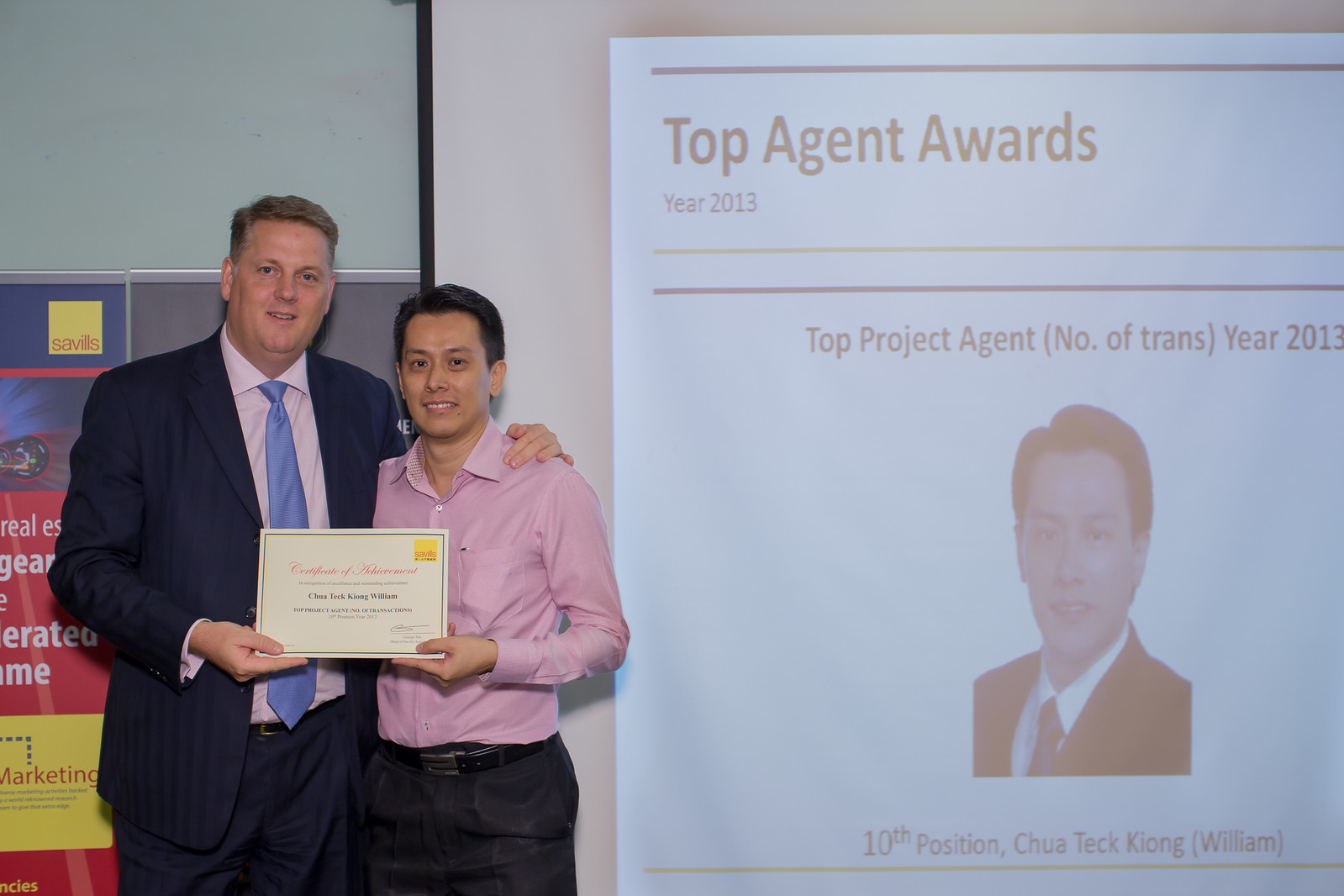The photograph captures a moment of recognition, featuring two men positioned on the left side of the frame. The man closest to the edge is a white man dressed in a navy blue suit, a pink shirt, and a light bluish-lavender tie, presenting a certificate to the second man, who appears to be of Asian descent, with dark black hair. The Asian man is wearing a rose-pink, long-sleeved button-down shirt paired with black dress pants and a black belt. Both men are jointly holding a small, tan-colored certificate, the text on which is too small to read. Behind them, partially visible on the left side, is a red sign with indistinct text. Dominating the background on the right is a projection screen that reads "Top Agent Awards Year 2013" and "Top Project Agent Number of Transactions Year 2013." The screen further identifies the Asian man as "Choi Taekyung William," who has achieved the 10th position, accompanied by a duplicate image of him receiving the award.